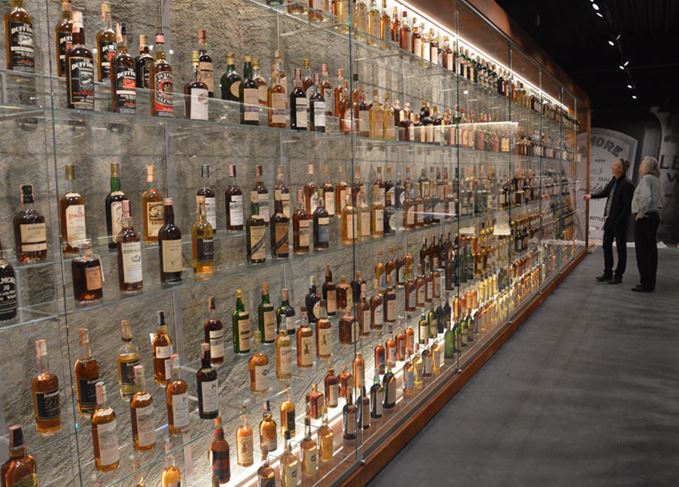This photograph captures a massive, well-lit display case spanning 20 to 30 feet, filled with hundreds of beautifully designed bottles of various alcohols. The display case, which features 9 to 10 glass shelves, forms an entire wall backed by stone, with wood paneling above and below. The bottles showcase a variety of labels and colored liquids from different manufacturers, and the carpeted room, possibly part of an alcohol museum or production plant, adds to the sophisticated ambiance. Two men dressed in formal black or gray outfits are visible in the top right corner, admiring the extensive and meticulously presented collection.